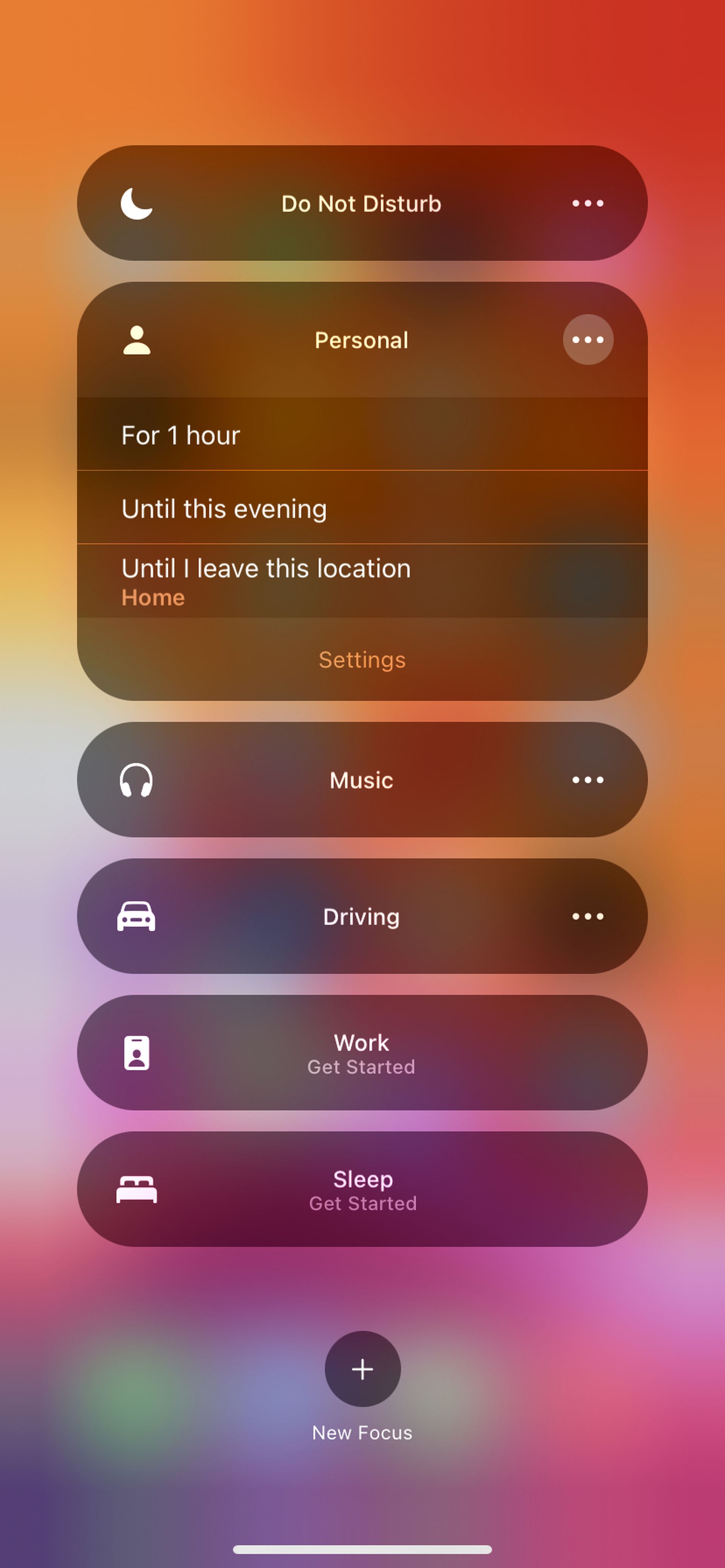This is a detailed screenshot of a smartphone's settings menu, displayed in a portrait orientation. The interface showcases various configuration options, organized into distinct sections represented by transparent black ovals stretching horizontally across the screen. Each section features an icon on the left and a settings indicator on the right.

1. **Do Not Disturb**
   - Icon: White moon symbol on the left.
   - Right: Three vertical dots indicating additional options.
   
2. **Personal**
   - Icon: Person symbol on the left.
   - Right: Three vertical dots indicating extra settings.
   - Options: "For 1 hour," "Until this evening," and "Until I leave this location – Home."

3. **Settings**
   
4. **Music**
   - Icon: Headphones symbol on the left.
   
5. **Driving**
   - Icon: Car symbol on the left.
   
6. **Work**
   
7. **Get Started**
   - Icon: Indistinct symbol resembling a book.
   
8. **Sleep**
   - Icon: Bed symbol on the left.
   - Right: "Get Started" option.
   
9. **New Focus**
   - Icon: Plus symbol on the left.

Each section allows toggling different settings, providing a streamlined and user-friendly approach to managing phone preferences and behaviors in specific contexts, such as sleep, work, and driving.